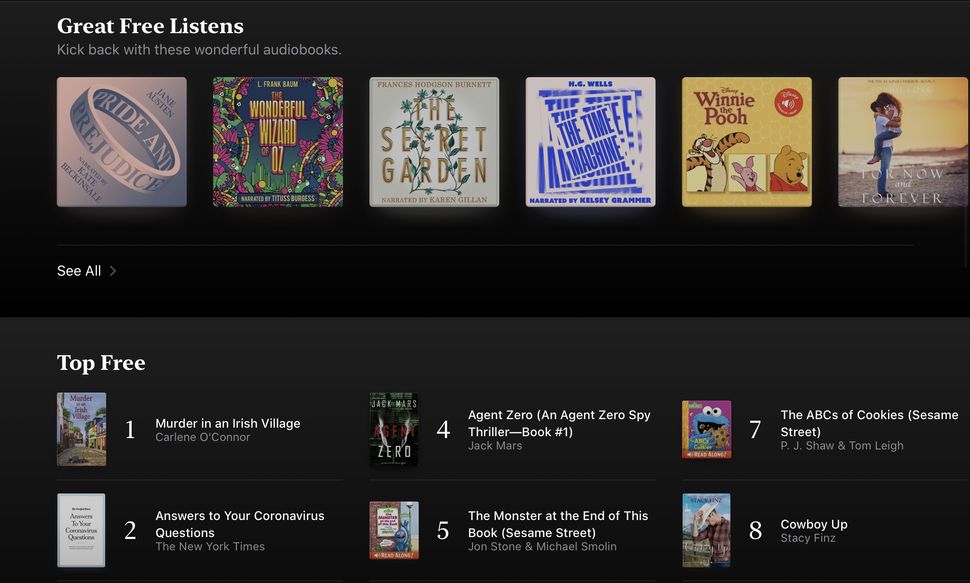Screenshot of a desktop or laptop showcasing a digital audiobook store or application. The interface has a sleek black background in widescreen landscape format, with bold white text that reads, "Great Free Listens: Kick Back with These Wonderful Audiobooks."

At the top, there's a carousel of featured audiobooks, each accompanied by a cover image. The titles include:

1. "Pride and Prejudice" by Jane Austen
2. "The Wonderful Wizard of Oz" by L. Frank Baum
3. "The Secret Garden" by Frances Hodgson Burnett
4. "The Time Machine" by H.G. Wells
5. "Winnie the Pooh"
6. "For Now and Forever"

Below the featured section, there's a "Top Free" category listing popular free audiobooks available:

1. "Murder in an Irish Village" by Carlene O'Connor
2. "Answers to Your Coronavirus Questions" by The New York Times
3. [Not Pictured]
4. "Agent Zero: An Agent Zero Spy Thriller, Book 1" by Jack Morris
5. "The Monster at the End of This Book: Sesame Street" by Jon Stone and Michael Smollin
6. [Not Pictured]
7. "The ABCs of Cookies: Sesame Street" by P.J. Shaw and Tom Leigh
8. "Cowboy Up" by Staci Finns

The clean and organized layout highlights a diverse selection of classic and contemporary audiobooks, perfect for all listening preferences.